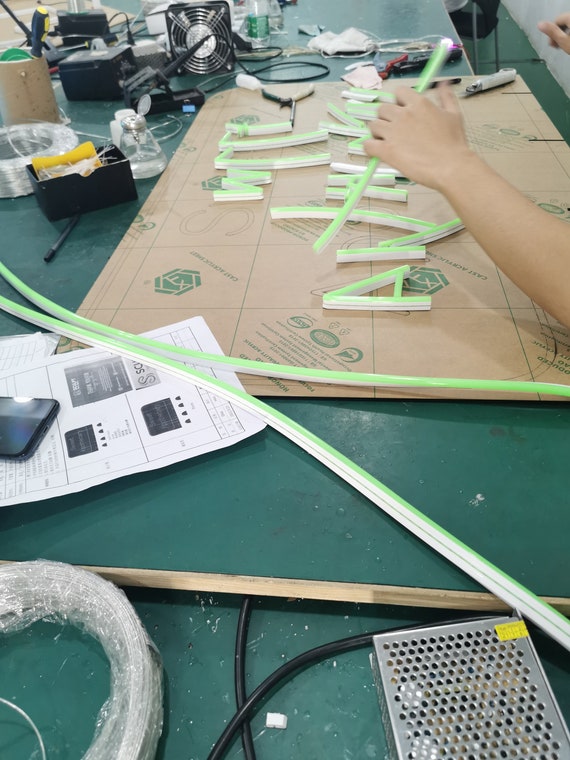In the photograph, a cluttered workstation is bustling with a project-in-progress. A long, dark green table holds an array of tools and materials, creating a vivid scene of meticulous handiwork. Prominently, two hands are busy shaping light green strips of material on a round piece of brown cardboard situated at the center. These strips appear to be plastic or foam, possibly intended to form letters such as 'W' and 'A'. The workspace is strewn with various items: a hot pen, a fan, glue, pincers, screwdrivers, a knife, pencils, a phone, tweezers, an array of cables, and even a stick. A set of instructions and a mobile phone lie nearby, indicating that the person is meticulously following guidelines to craft what resembles an LED sign. The image captures the essence of a dedicated craftsperson deeply engrossed in their detailed work amidst a lively, tool-laden table.